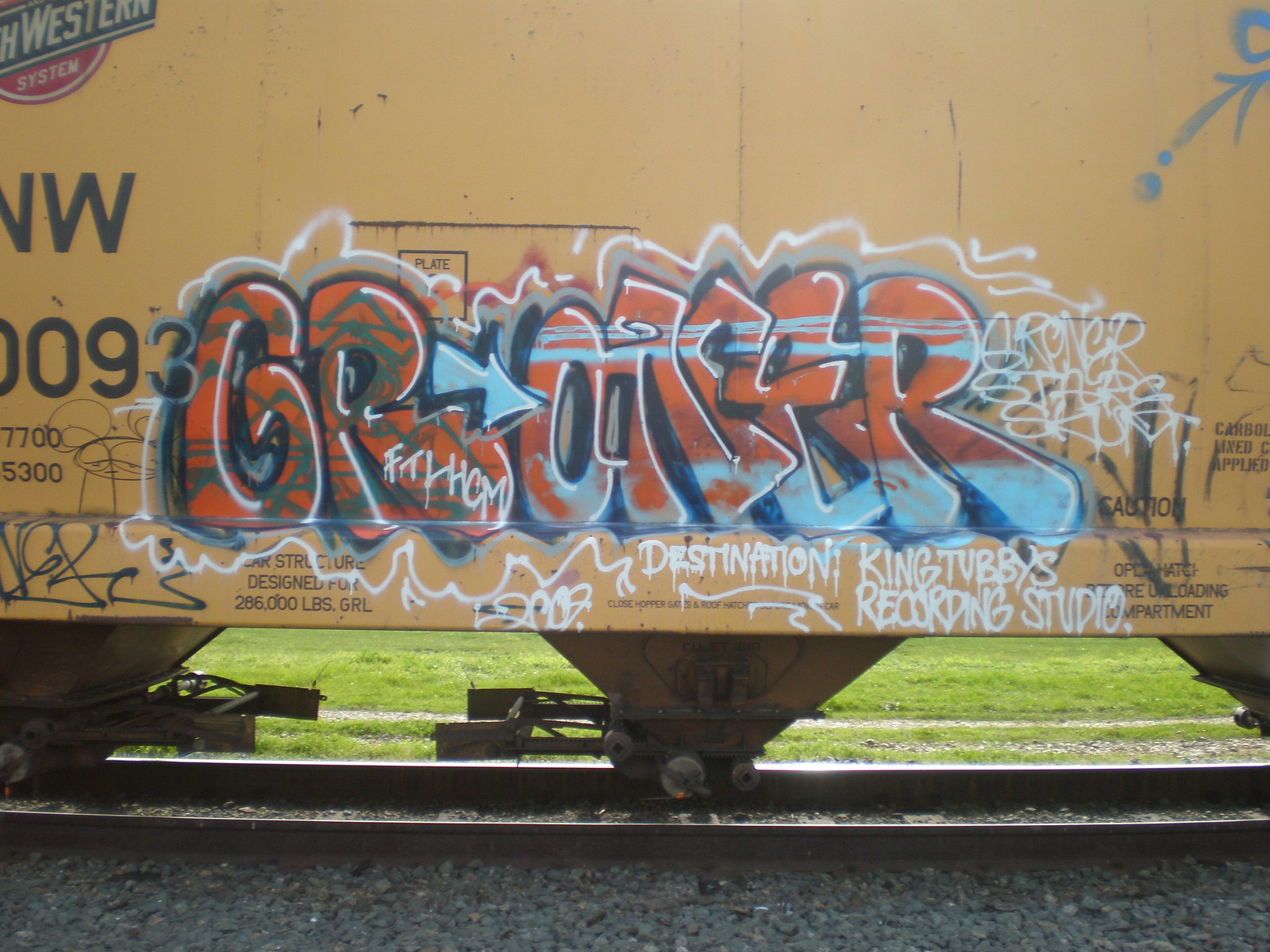This outdoor image showcases the side of a yellow train car adorned with vibrant graffiti. The graffiti features bubble-like, 3D uppercase letters predominantly in green and orange, with accents of blue and white splashed through them. Among the graffiti, the word "destination" stands out, along with "King Tubby's Recording Studio," and the cryptic "G something scum" (S-K-U-M). Additionally, a blue arrow is painted on. In the bottom corner of the car, the words "Northwestern System" and "NW-0093" are marked. The train car, covered with various manufacturer stamps such as "designed by" and "286 pounds," rests on steel rails surrounded by gravel, with some grass visible in the background.